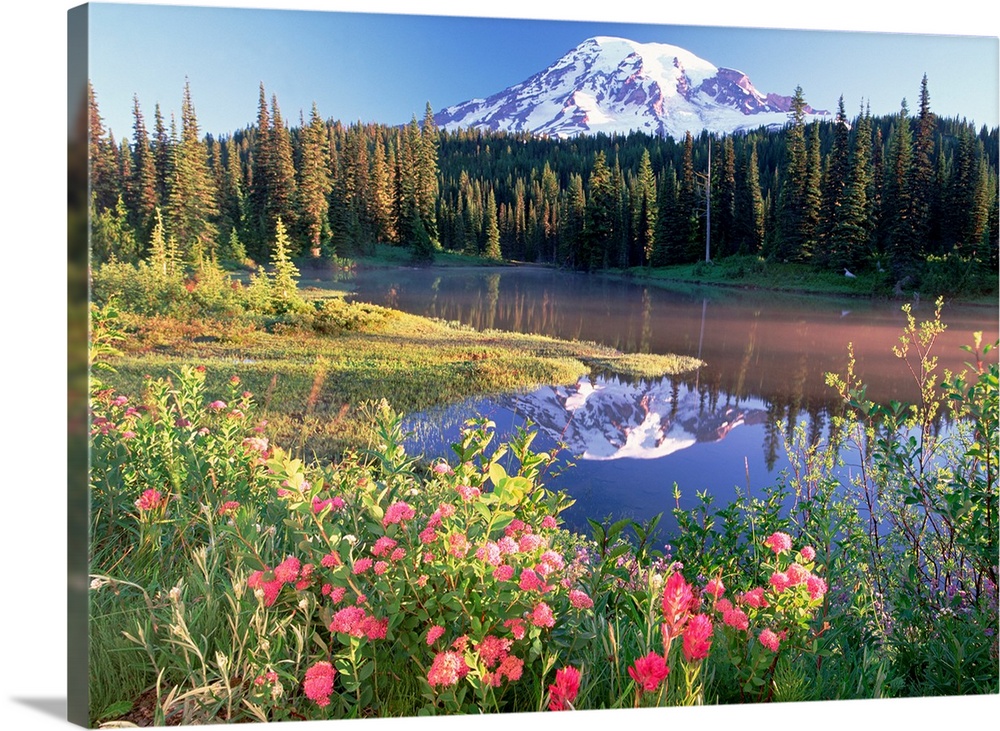The image captures a breathtaking mountain scene on a bright, sunny day, showcasing a majestic snow-capped mountain that appears slightly brownish-red due to the sunlight and distance. The mountain, towering in the background, contrasts beautifully with the crisp blue sky above and is reflected in a serene river or lake below. At the base of the mountain lies a dense forest of vibrant green evergreen trees set against patches of red trees. The water in the foreground subtly shifts in color, appearing red where it catches the sun's rays and blue in its depths, mirroring the snowy peak perfectly. In the immediate foreground, a lush area adorned with pink, purple, and green flowers interspersed with grass and vegetation adds a splash of color and texture to the scene, creating a vivid and harmonious natural landscape.